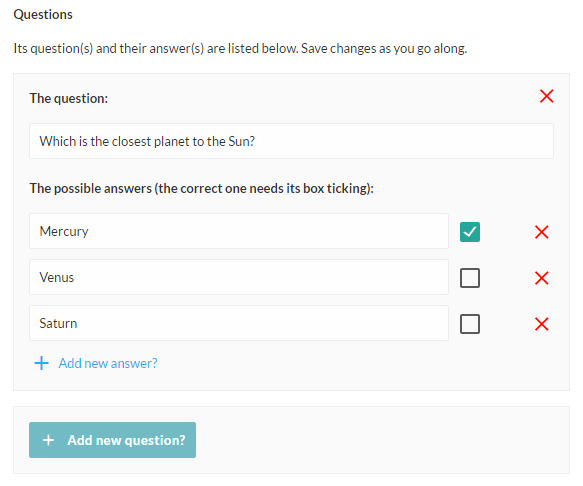The image showcases a form designed for setting up questions and answers. At the top, the word "Questions" is prominently displayed in bold text. Beneath this heading, there's an instruction indicating that questions and their corresponding answers are listed below, along with a reminder to save changes as you go.

The form starts with the question "Which is the closest planet to the Sun?" followed by a rectangular text box for inputting this specific question. Below the question, "Possible Answers" is highlighted in bold text, with instructions that the correct answer should be marked by ticking its corresponding box.

Three rectangular boxes follow, each containing a possible answer: "Mercury," "Venus," and "Saturn." To the right of each box is a small square checkbox; the box next to "Mercury" is checked, indicating it as the correct answer. Both the question and each answer option include a red 'X' on their right side for removal purposes.

Additional functionalities are provided below the answers. There is a small blue plus sign reading "Add new answer," allowing for the insertion of more than three possible answers. At the bottom, a green button with white text and a plus sign is available, marked "Add new question," to facilitate the addition of further questions.